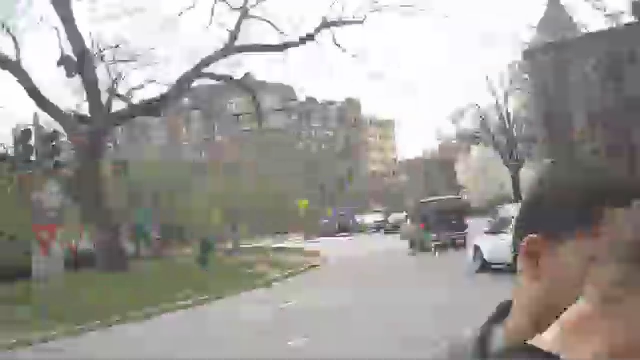This low-quality, grainy image captures a street scene bordered by apartment-like buildings in the background. The street is lined with a series of parked cars. In the foreground at the bottom right corner, a side profile of a person with blonde hair can be seen, though their face is cut off by the image's margin. Slightly behind them, partially obscured, is another individual with short brown-black hair, only their ear, cheek, and neck visible. To the left bottom of the image, a small patch of green grass is visible accompanied by a tall, leafless tree, anchoring the scene in a bleak, possibly autumn, or early winter setting.